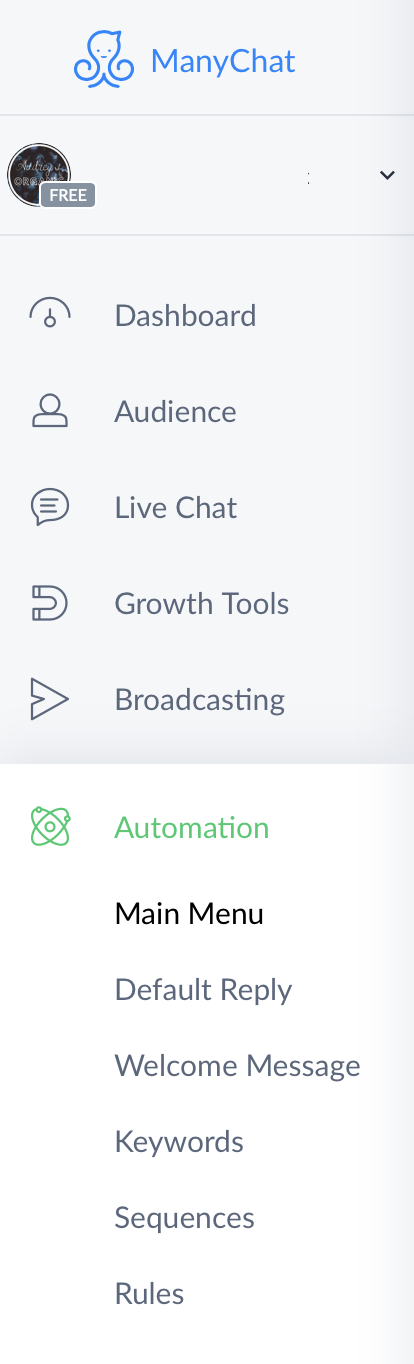The image is a vertical, rectangular screenshot from an application interface. At the top, there is a blue logo featuring a simplistic line drawing of an octopus-like creature with two dots for eyes, a small line for a mouth, and a pointed appendage extending from its head. Next to this logo, also in blue, is the text "ManyChat" in uppercase letters. Beneath the logo, a gray horizontal line separates the header from the rest of the interface.

Below this line, there is an oval shape which appears to be a placeholder for a profile picture, although the image within it is unreadable. Alongside the profile picture, the word "Free" is marked, indicating a free plan or subscription. Adjacent to this, there is a pull-down menu featuring options listed in gray text: "Dashboard," "Audience," "Live Chat," "Growth Tools," and "Broadcasting."

Continuing downward, against a lighter gray background, additional menu items are listed: "Automation," "Main Menu," "Default Reply," "Welcome Message," "Keywords," "Sequences," and "Rules." These options appear to be part of the navigation or settings within the application. The overall design is minimalist, utilizing varying shades of gray to distinguish different sections and menu items.